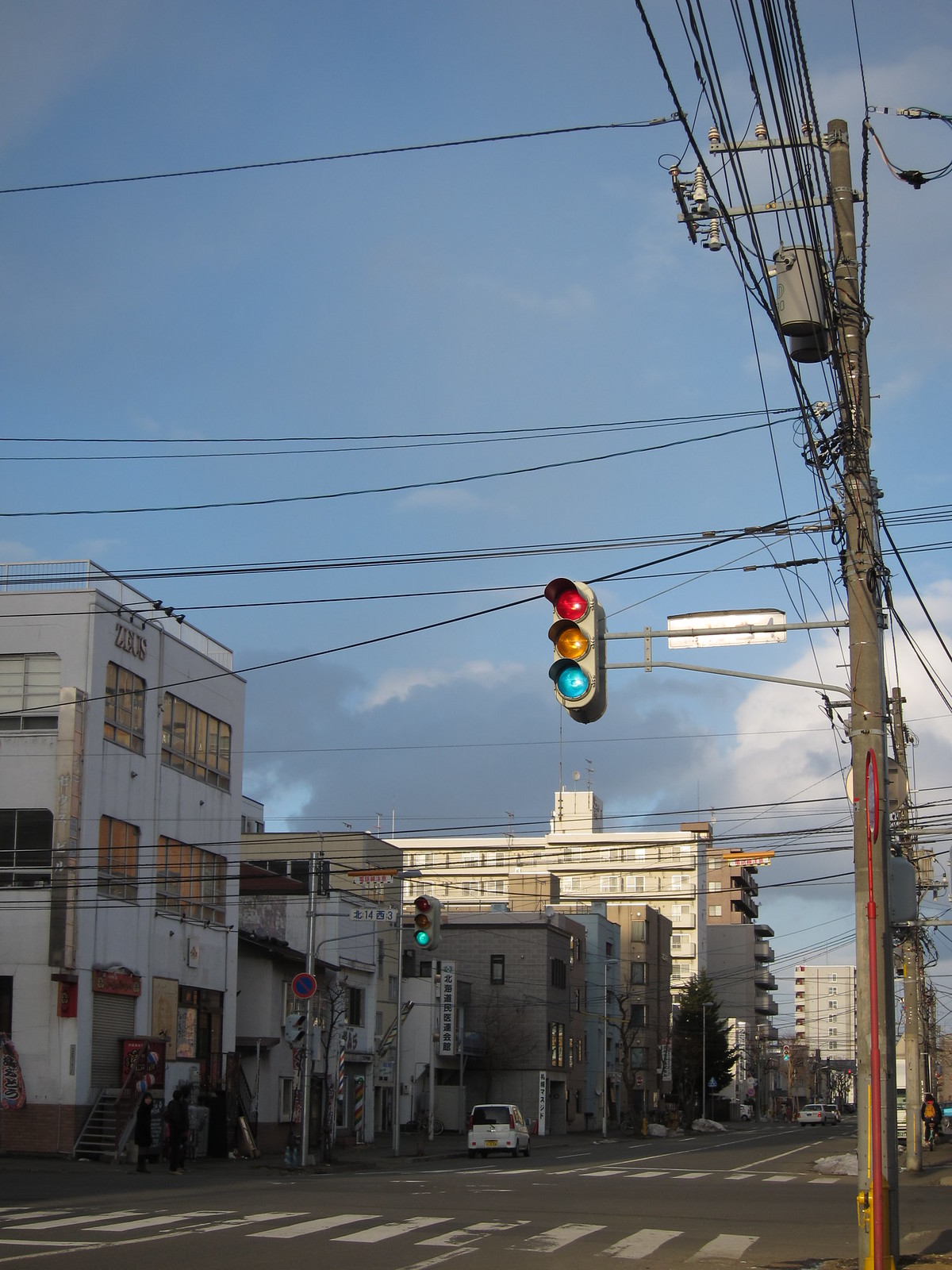This photograph captures a bustling urban neighborhood that likely resides in Japan or China, evident from the Asian letters adorning the buildings. The image showcases a mix of two to three-story residential structures in the foreground, with taller condominium or high-rise apartment buildings, approximately 8 to 12 stories high, standing in the background. The scene unfolds at an intersection marked with crosswalks and street lights, one of which currently displays a green signal.

The sky above is a mix of light blue hues and large gray clouds, casting a soft light over the landscape. Prominent in the foreground are large power poles and telephone poles, festooned with an intricate web of black and gray electric and transmission wires that crisscross above the street. The buildings in this neighborhood are primarily light-colored, featuring shades of tan, cream, white, and some brickwork.

The street itself is a blacktop road, bordered by cars parked along the sides, and a distant white car can be seen further down the road. Two people, dressed in black clothes, walk along the sidewalk. The presence of traffic signs and stoplights, vividly showing red, yellow, and green lights, further emphasizes the urban setting. The scene encapsulates the essence of a lively, residential district amidst a bustling cityscape.